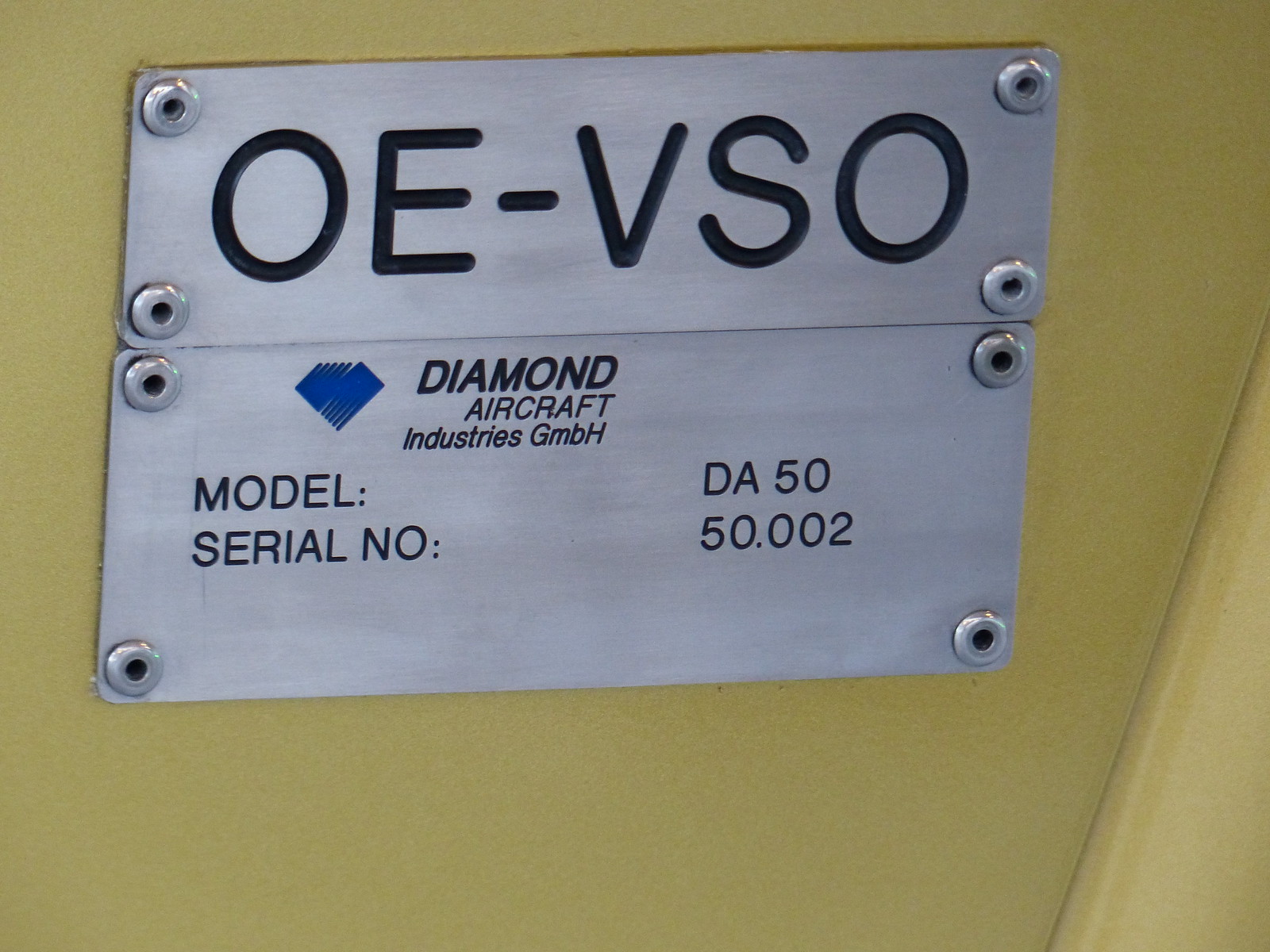The image depicts a silver metallic plate bolted onto a mustard yellow surface with a total of eight rounded bolts, four on each side. The plate features several inscriptions in black lettering. At the top, in large letters, it reads "OE-VSO." Below this, there is a blue diamond logo created with diagonal lines. To the right of the logo, the plate is inscribed with "Diamond Aircraft Industries GMBH" in italicized black letters, with the 'G' and 'H' capitalized. Further down, the left side of the plate denotes "Model" and "Serial Number," while the corresponding details "DA-50" and "50.002" are listed on the right side. The metallic object appears slightly aged and worn, contributing to the overall rugged look of the label.